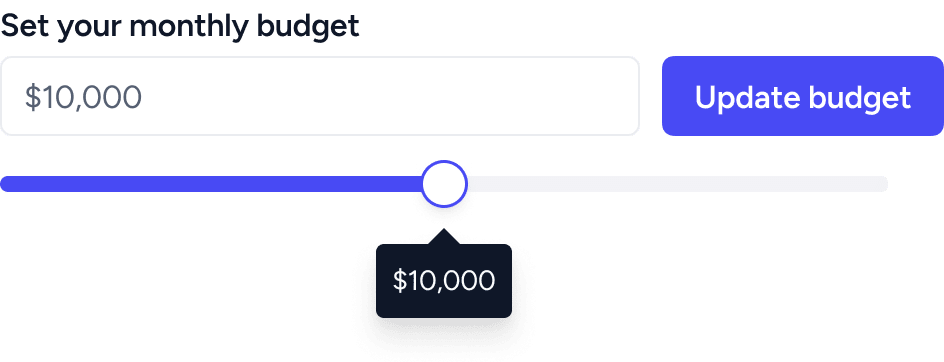A focused screenshot of a budgeting control panel from an unidentified app. The interface features a minimalist design centered around a section labeled "Set Your Monthly Budget" in soft, rounded, black sans-serif font located in the upper left corner. Directly below this text, a user-input field displays a budget of "$10,000." To the right of this field is a prominent purple button with white text stating "Update Budget," designed with a rectangular shape and rounded corners for a modern aesthetic.

Below the input field lies an interactive slider. The slider consists of a blue bar extending to the left, a white circle edged with a thin blue line in the middle, and an empty bar to the right of the circle. Directly beneath this slider, a downward-facing speech bubble displays the budget value "$10,000" in white text against a very dark gray or black background, emphasizing the selected budget amount.

The overall background remains plain white, accentuating the functionality elements within this narrow, wide screenshot, highlighting that it’s a specific part of the app rather than a full view of the application or website. This particular screen is clearly designed to allow the user to set and update their initial budget, likely a preliminary step before engaging with the app’s full suite of budgeting tools and features.